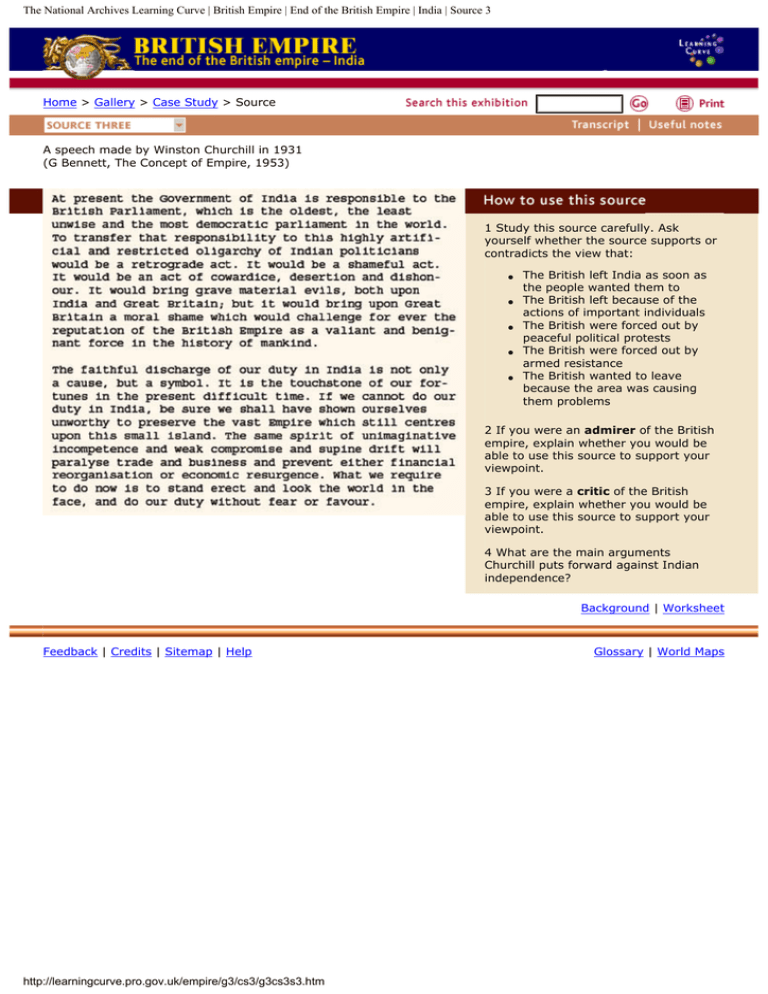Caption: 

This image depicts a webpage from The National Archives' Learning Curve series, focusing on the End of the British Empire in India. The website's color scheme is predominantly white, beige, and blue, with red accents and mostly black text. At the top of the page, a white bar displays the title "The National Archives Learning Curve" followed by "British Empire, End of the British Empire, India, Source 3." Below is a blue bar with "British Empire" written in yellow, and to the right, "Learning Course" is visible in the far-right corner. An icon resembling a globe is positioned next to the "British Empire" text. 

Underneath this, a red bar contains navigation options including "Home," "Gallery," "Case Study," and "Source." A "Search this Exhibition" section is present with a search box, a "Go" button, and a "Print" button. Further down the page, a box allows users to click through more sources; currently, "Source 3" is selected. 

Buttons for "Transcript" and "Useful Notes" are visible. To the right, a detailed description on how to use the source is provided. The left side displays the source itself: a speech made by Winston Churchill in 1931, cited from G. Bennett’s "The Concept of Empire" (1953). The speech begins, "At the present, the government of India is responsible to the British Parliament, which is the oldest, the least unwise, and most democratic parliament in the world," and continues with two paragraphs of text. 

The right panel offers guidance on how to analyze the source, including a prompt to assess if the source supports or contradicts certain views, followed by bullet-pointed instructions. Additional buttons for "Background," "Worksheet," "Glossary," "World Maps," "Feedback," "Credits," "Sitemap," and "Help" are highlighted in blue across the page.